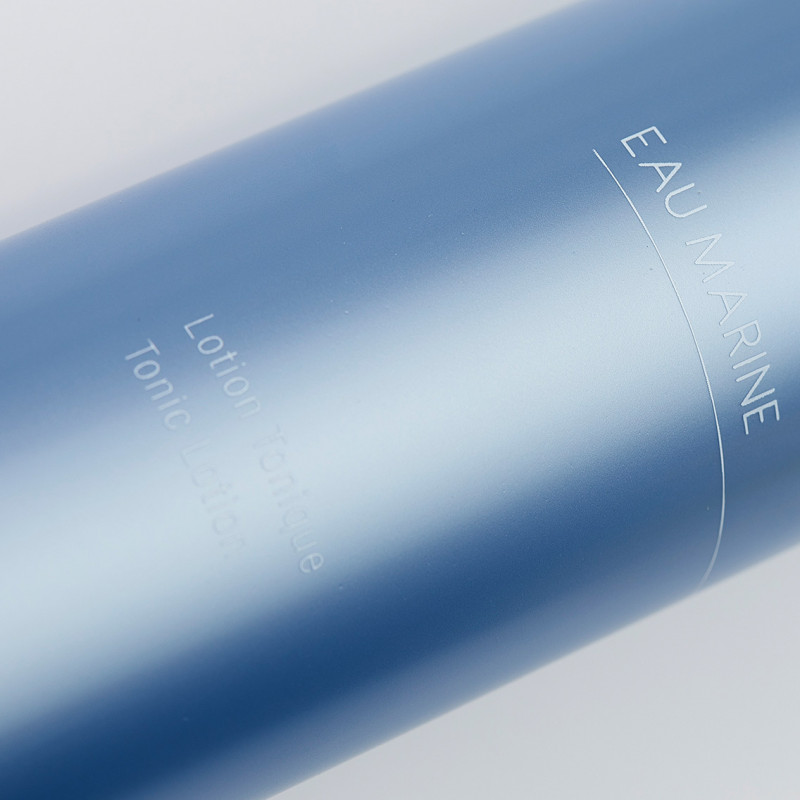This is an extreme close-up image of a cylindrical plastic container, likely a lotion bottle, set against a medium gray background. The bottle is tilted diagonally, running from the lower left-hand corner to the upper right-hand corner of the frame. Its surface displays a gradient of steel blue to almost white where the light hits it, creating a white reflection down the center that makes some of the text difficult to read. The label reads "O Marine" or "E-Marine" at the top in prominent white text, followed by smaller descriptive text. Towards the bottom, the terms "lotion tonique" and "tonic lotion" can be seen, albeit partially obscured by the bright reflection. The overall image is slightly blurry or out-of-focus, giving it a soft-focused appearance that emphasizes the container's color gradient and text details.